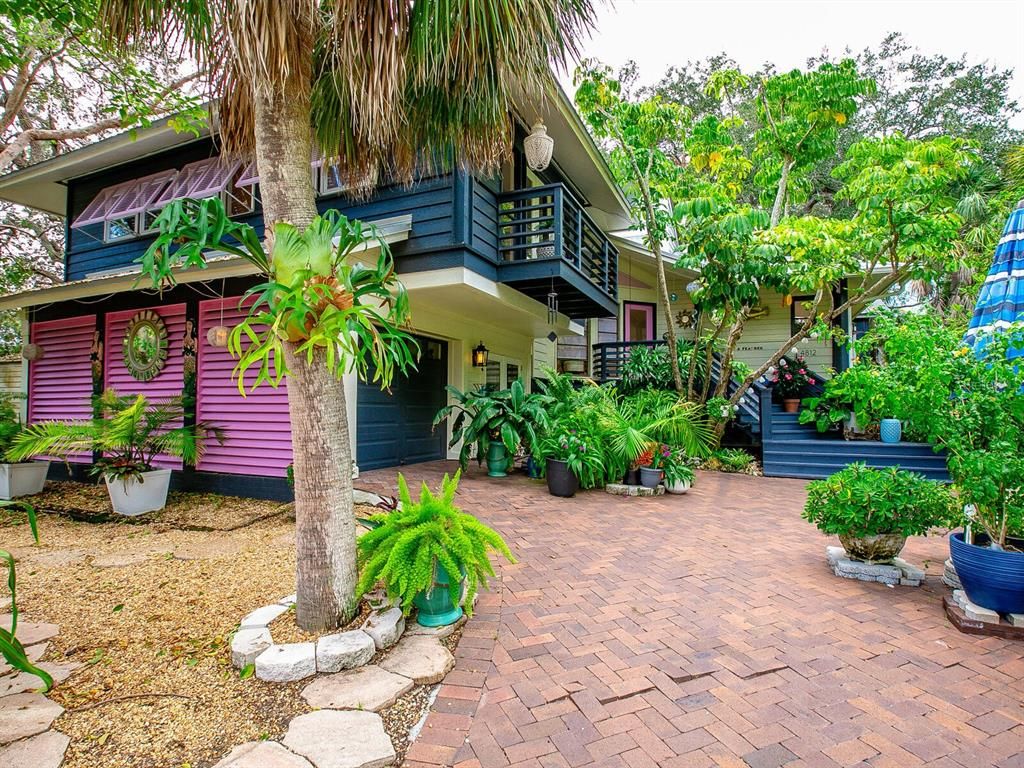This vibrant photograph captures a charming, colorful two-story home set in a tropical location, perhaps somewhere like Florida or Louisiana. The house features a striking mix of dark blue, white, and vivid fuchsia accents. Its distinctive façade has a deep blue balcony above a one-car garage, with matching blue steps leading up to the main entrance, which is outlined in fuchsia. The windows and shutters are a cheerful lilac color, lending a playful, welcoming feel to the house.

The driveway, composed of herringbone-patterned brick pavers, shows signs of wear with visible cracks in the foreground. To the left of the driveway, a tall palm tree and several other tropical plants signal the lush, humid environment. Numerous potted plants, including bright green ferns and other large tropical varieties, are scattered throughout the property, adding to the vibrant and lively atmosphere. The pristine, clear, sunny sky enhances the overall brightness and cheerful ambiance of this well-loved home.